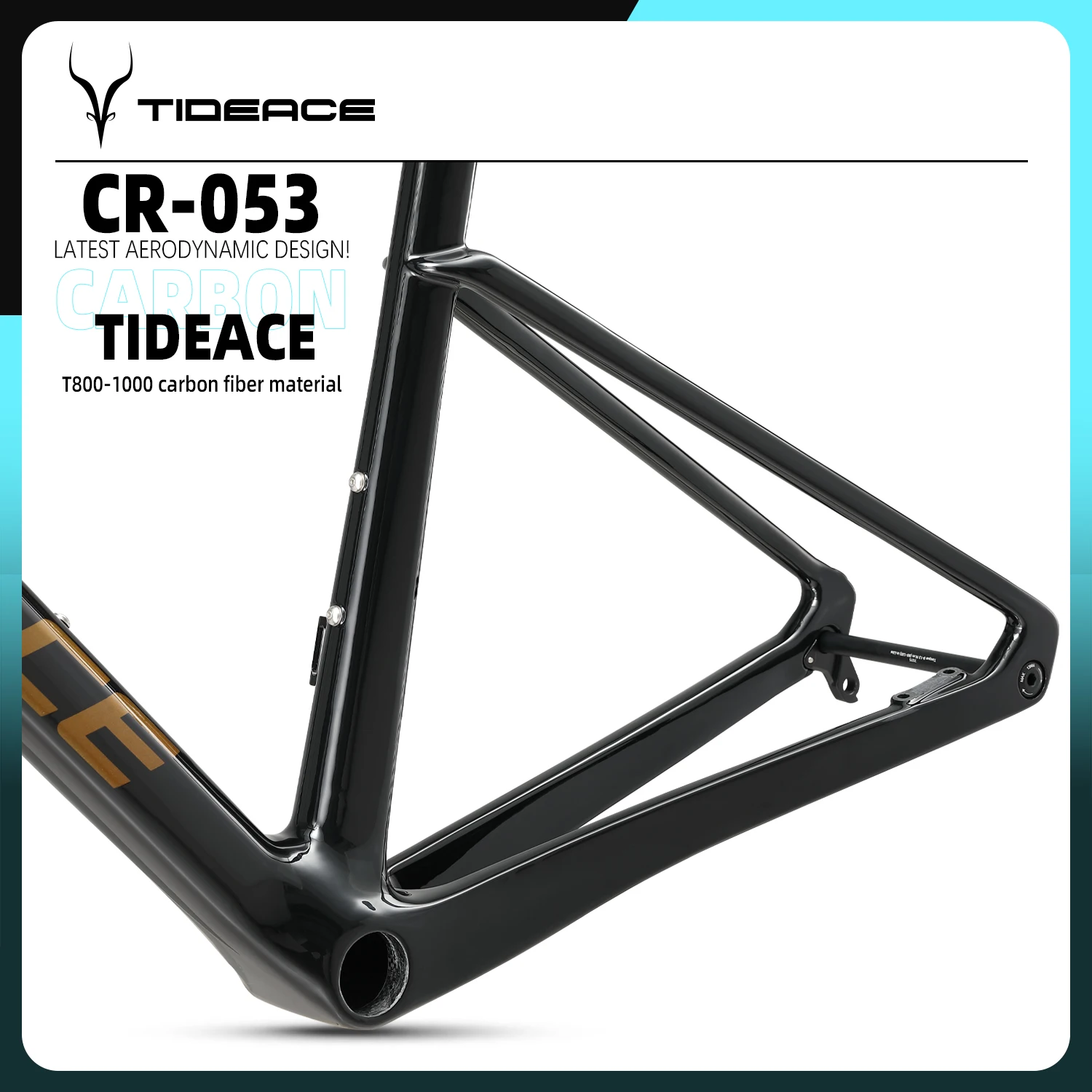The advertisement features a detailed and professional photo of what appears to be a bicycle frame, specifically a model CR-053 from TIDEACE, crafted with advanced T800 to 1000 carbon fiber material renowned for its latest aerodynamic design. Positioned within a box that has a distinctive border transitioning from black in the top left corner to shades of blue and slate, the ad is both visually striking and informative. In the top left corner, there's a logo resembling antlers with the brand name "TIDEACE" beside it in black. Below the logo, a straight black line runs horizontally, followed by the text "CR-053 latest aerodynamic design carbon TIDEACE T800-1000 carbon fiber material," emphasizing the high-quality construction of the product. The showcased gray V-shaped metal piece, with additional V-shaped extensions, underscores the sleek and innovative design of the bicycle frame. The ad's border, alternating between black and aqua, frames the image against a white background, enhancing the image's professional aesthetic. The advertisement also directs viewers to visit www.Flydreamers.com for more information.